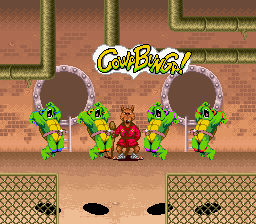In this detailed screenshot from a computer game, the background features a light orange hue, creating a warm and inviting atmosphere. The lower part of the scene is colored in brown, grounding the environment. At the center of the image stands a prominent character with a distinct brown head, adorned in a striking red and yellow robe, capturing the eye.

Flanking the central character are four Ninja Turtles, two positioned on each side. The turtles stand against a background wall marked by dark brown circular designs, which are outlined in lilac, adding a subtle decorative touch.

In the lower left and right corners of the image, there are intricate brown lattice patterns, giving a textured feel to the scene. Spanning horizontally along the bottom of the frame are several oval-shaped black forms, perhaps representing shadows or additional elements of the game’s design.

Emerging from the top of the image are green pipes, reminiscent of classic video game elements. On the left side, a backward L-shaped pipe directs attention inward. At the center, a long L-shaped pipe stretches down, and just above it, another long pipe, slightly shorter in length, adds to the vertical complexity of the layout. Together, these elements craft a visually engaging and multifaceted game scene.